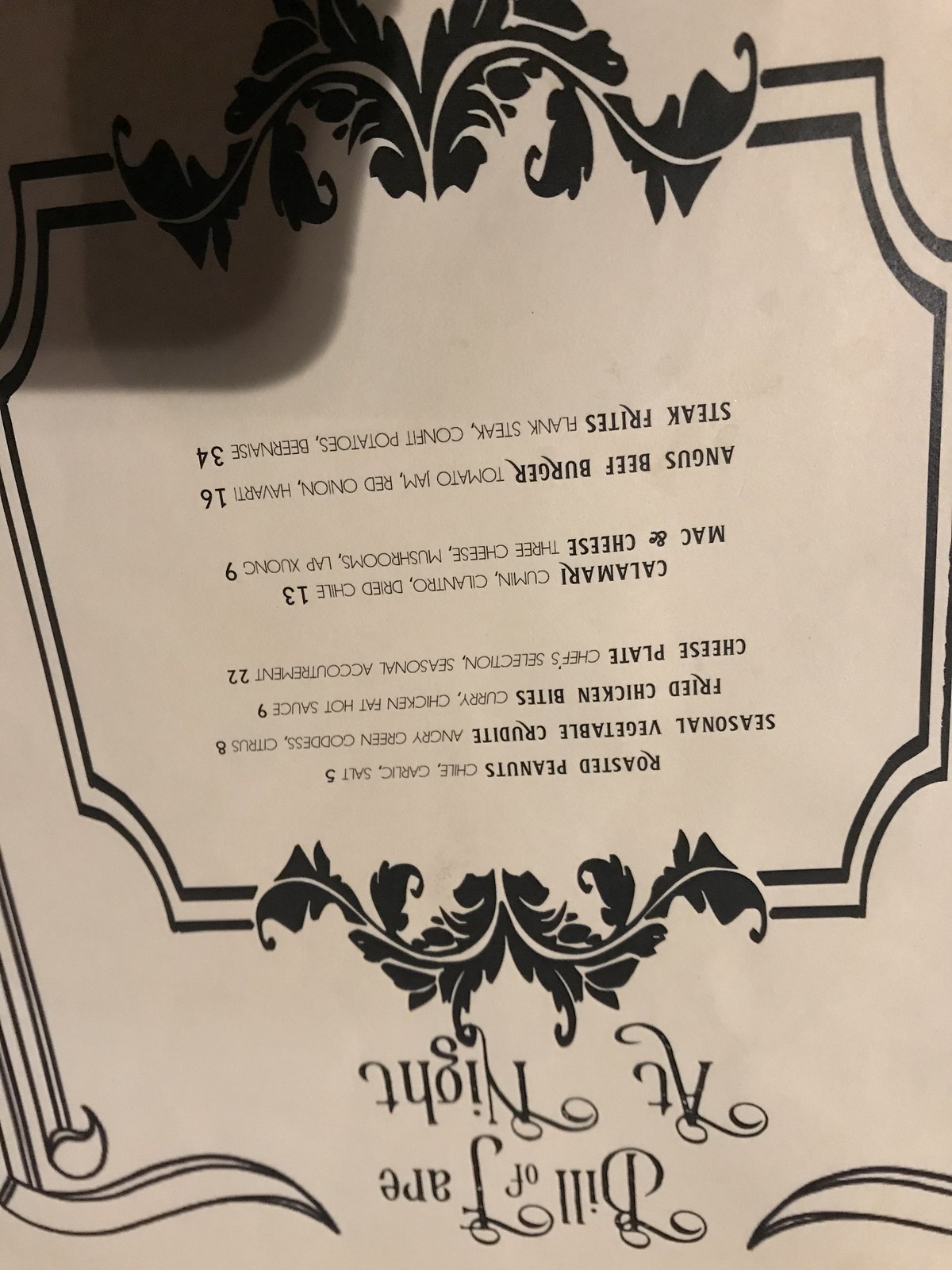This image is an upside-down menu showcased on an off-white background adorned with black line and floral designs around its edges. The title at the top reads "Bill of Fare at Night," followed by a list of menu items detailed in descending order.

From top to bottom and left to right, the menu items include:
- Roasted Peanuts with chili, garlic, and salt for $5.
- Seasoned Vegetable Crudités described with additional text, priced at $8.
- Fried Chicken Bites with a description mentioning curly chicken and hot sauce, priced at $9.
- Cheese Plate with a lighter-colored, hard-to-read description, priced at $22.
- Calamari for $13.
- Mac and Cheese for $9.
- Angus Beef Burger for $16.
- Steak Frites for $34, each accompanied by a corresponding description.

A slight dark shadow is noticeable in the top left corner of the image.